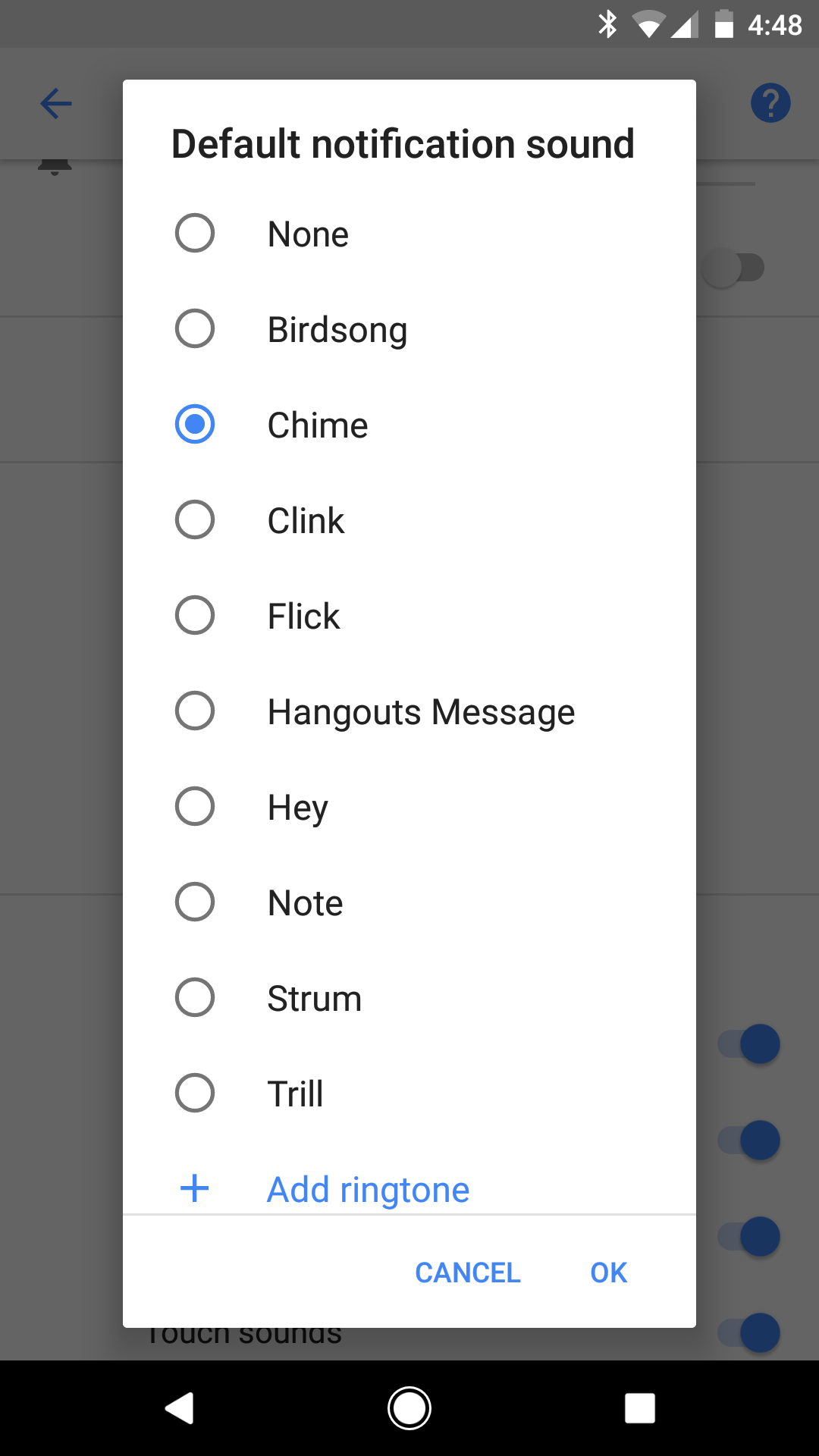The image is a digital screen capture of a cellphone's settings interface, specifically focusing on the "Default Notification Sounds" section. At the center of the screen is a white rectangular pop-up window. At the top of this window, the title "Default Notification Sounds" is prominently displayed.

Below the title is a column of various sound options, each accompanied by a radio button on the left. There are about six or seven options visible in this column. The third option, labeled "Chime," is selected, indicated by a blue dot within its radio button. Other visible sound options include "None," "Birdsong," "Click," "Flick," "Hang-out Message," "Hey," "No," "Strum," and "Thrill."

At the bottom of the column, there is an additional option labeled "Add Ringtone," followed by buttons for "Cancel" and "OK." The selected options — "Chime," "Add Ringtone," "Cancel," and "OK" — are highlighted in blue for emphasis. The font for all text remains black, ensuring clarity and readability.

The background image of the cellphone is grayed out, which serves to highlight the pop-up window and draw attention to its content. This layout aims to guide users through the process of setting their default notification sound, effectively illustrating how to select the "Chime" option.

Overall, the screen capture functions as a step-by-step visual guide to help users navigate the settings to customize their notification sounds on a cellphone.